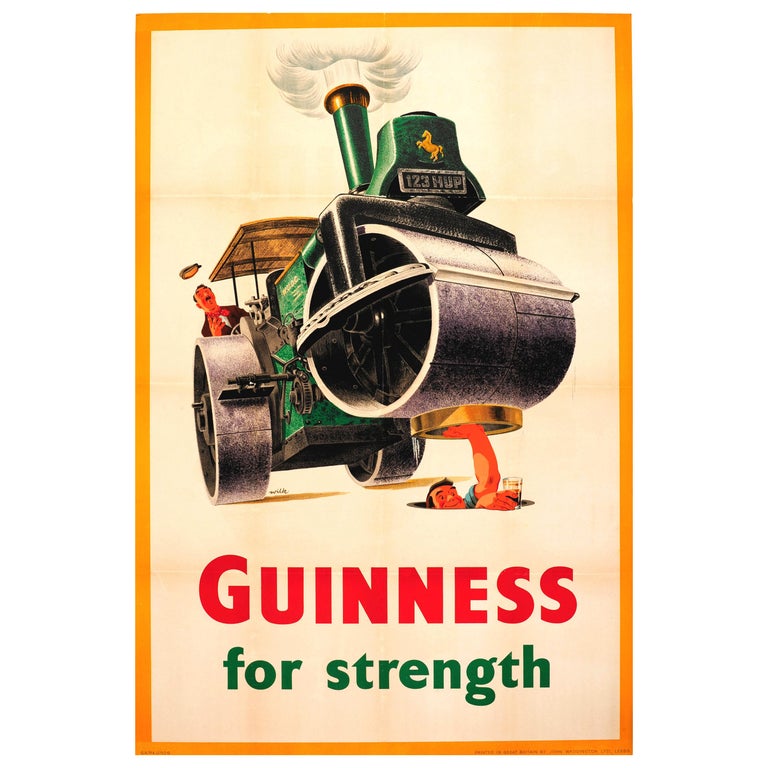The image is an old Guinness beer advertisement in a vertical rectangle format, featuring an eye-catching orange border. At its center, a green steamroller with a large gray roller at its front dominates the scene. The steamroller, which subtly faces to the right, has a small smokestack emitting a puff of white smoke in a circular shape. Notably, a man is emerging from beneath the steamroller's massive front roller through a manhole, showcasing his impressive strength by lifting the roller with one arm. The man, whose skin is depicted as orange, holds a glass of brown liquid—presumably Guinness beer—in his other hand. At the helm of the steamroller is an astonished driver, partially shielded by a small overhang at the back of the driver's area. The green steamroller features a distinctive gold or yellow horse decal on its front, adding to its unique design. Underneath this vivid scene, the words "Guinness" appear in bold red letters, followed by "for strength" in slightly smaller green letters, emphasizing the beer's empowering quality.